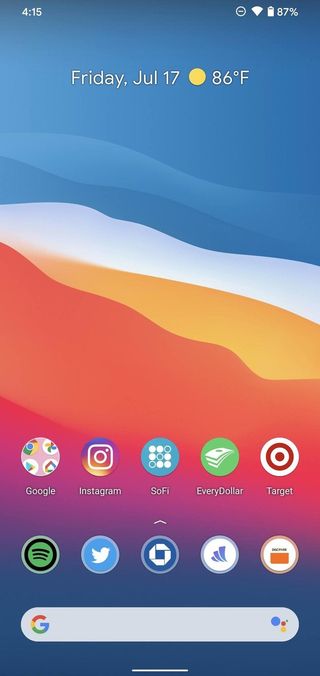This image is a detailed screenshot of a mobile device's home screen, taken at 4:15. The top left corner displays the time, while the top right corner shows essential status icons: a Wi-Fi symbol, a do-not-disturb icon (minus symbol within a circle), and a battery icon with an 87% charge. The background features a vibrant, wavy color pattern ranging from blue, light blue, white, yellow, red, peach, orange, pink, and dark navy blue at the bottom.

The home screen is organized with app icons and information. At the very top, the date "Friday, July 17th" is displayed alongside the weather, indicating a temperature of 86°F. Below this, an array of app icons is arranged. The first row includes a folder labeled "Google," Instagram, SoFi (a banking app), EveryDollar, and Target. The second row contains Spotify, Twitter, two unclear blue and white icons that potentially include the Citibank app, and an icon for Discovery. At the very bottom of the screen lies the Google search bar, completing the layout of this mobile device's home interface.